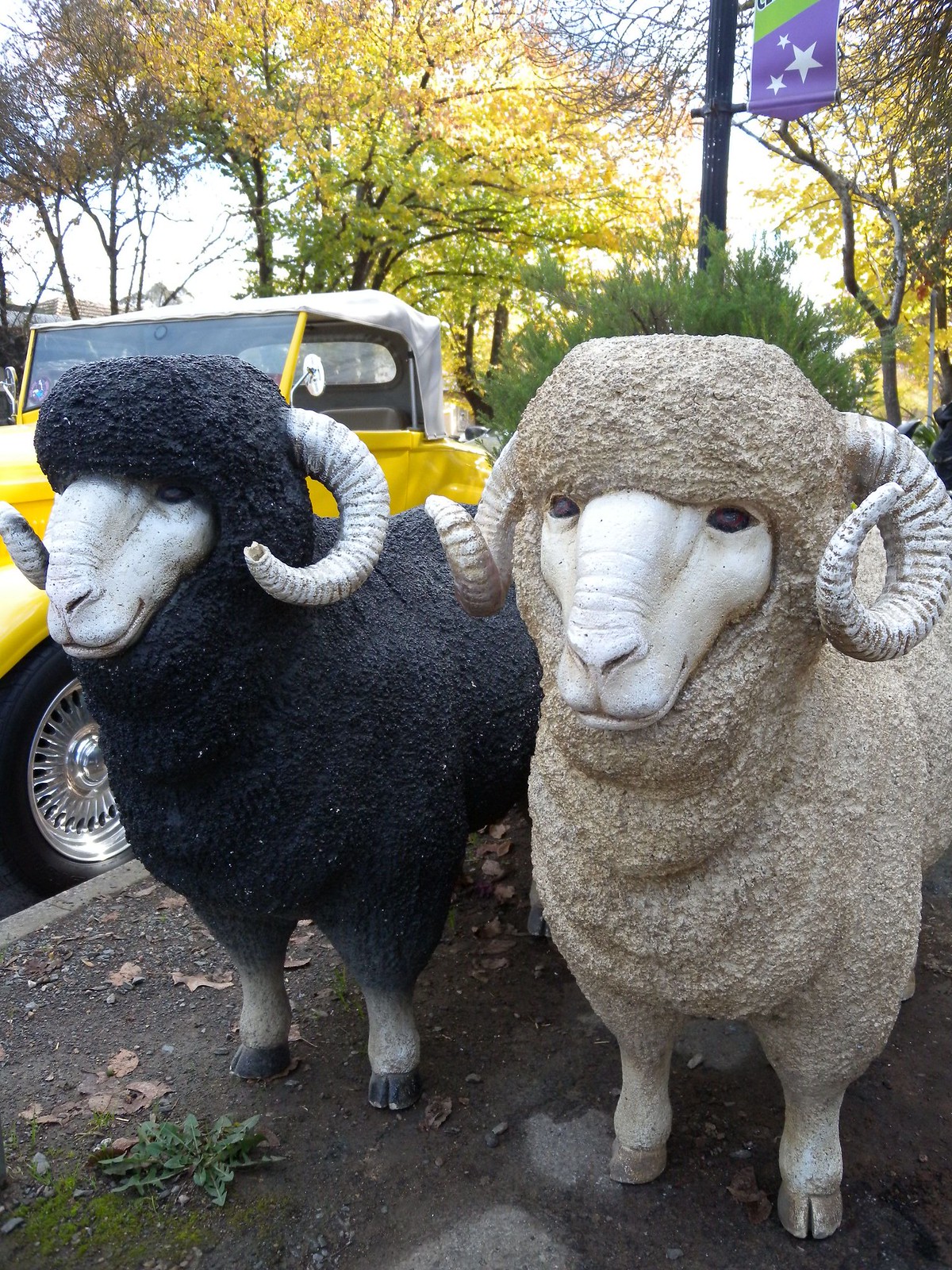This photograph features two detailed statues of bighorn sheep. The statue situated closer to the photographer has a cream-colored body, matching cream horns, and black eyes, while the one slightly further to the right is adorned with black wool, a cream face, white horns, and also black eyes. Both statues possess neutral, calm expressions and stand on a slightly damp, brown dirt surface. A small green plant can be seen in front of them. To the left in the background, partly obscured by the statues, there is a yellow car with fancy rims, likely a convertible with a cloth top. Further behind, a light pole rises alongside various trees, whose green, brown, and yellow leaves are visible against the blue sky. A green and purple flag is also partially seen waving in the background, adding to the scene's outdoor ambiance.